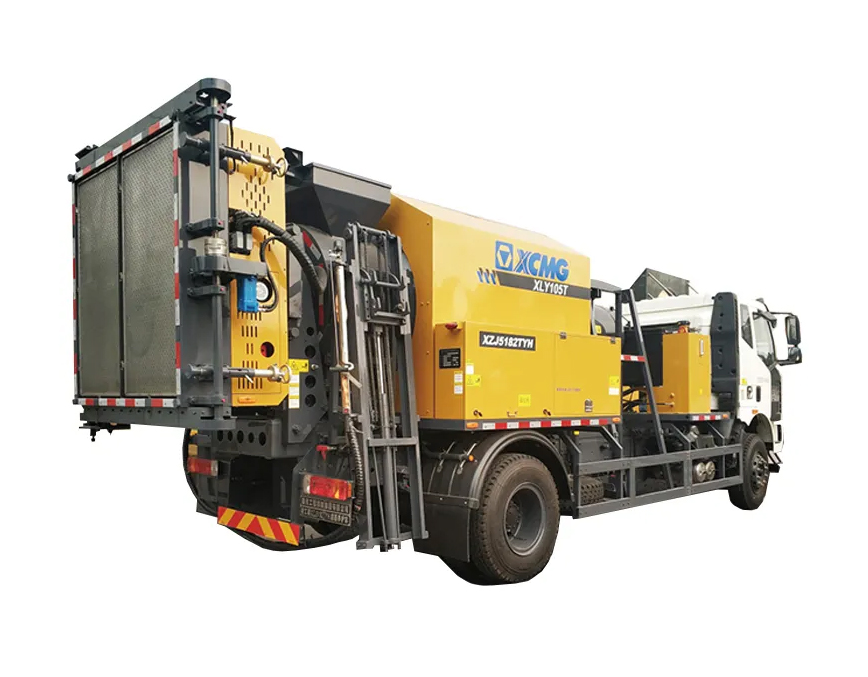The photograph depicts a large industrial truck predominantly used for construction purposes. The truck features a distinctive yellow side with the brand name "XCMG" prominently displayed. Below the brand name on the left side of the truck, there are two gray rectangles, one stating "XLY105T" and the other "XZJ5182TYM." The vehicle has black tires and a red and gold panel, and is equipped with a black back door. The truck's front part is white, including the driver's cockpit, which also features reflective mirrors. The image captures the back of the truck on the left and the front extending far to the right, emphasizing its significant size. There is a ladder attached to the truck, likely intended for access to higher areas of the vehicle. Overall, the truck is marked with various brown details and red and white trim, making it well-suited for heavy-duty tasks typically found at construction sites.